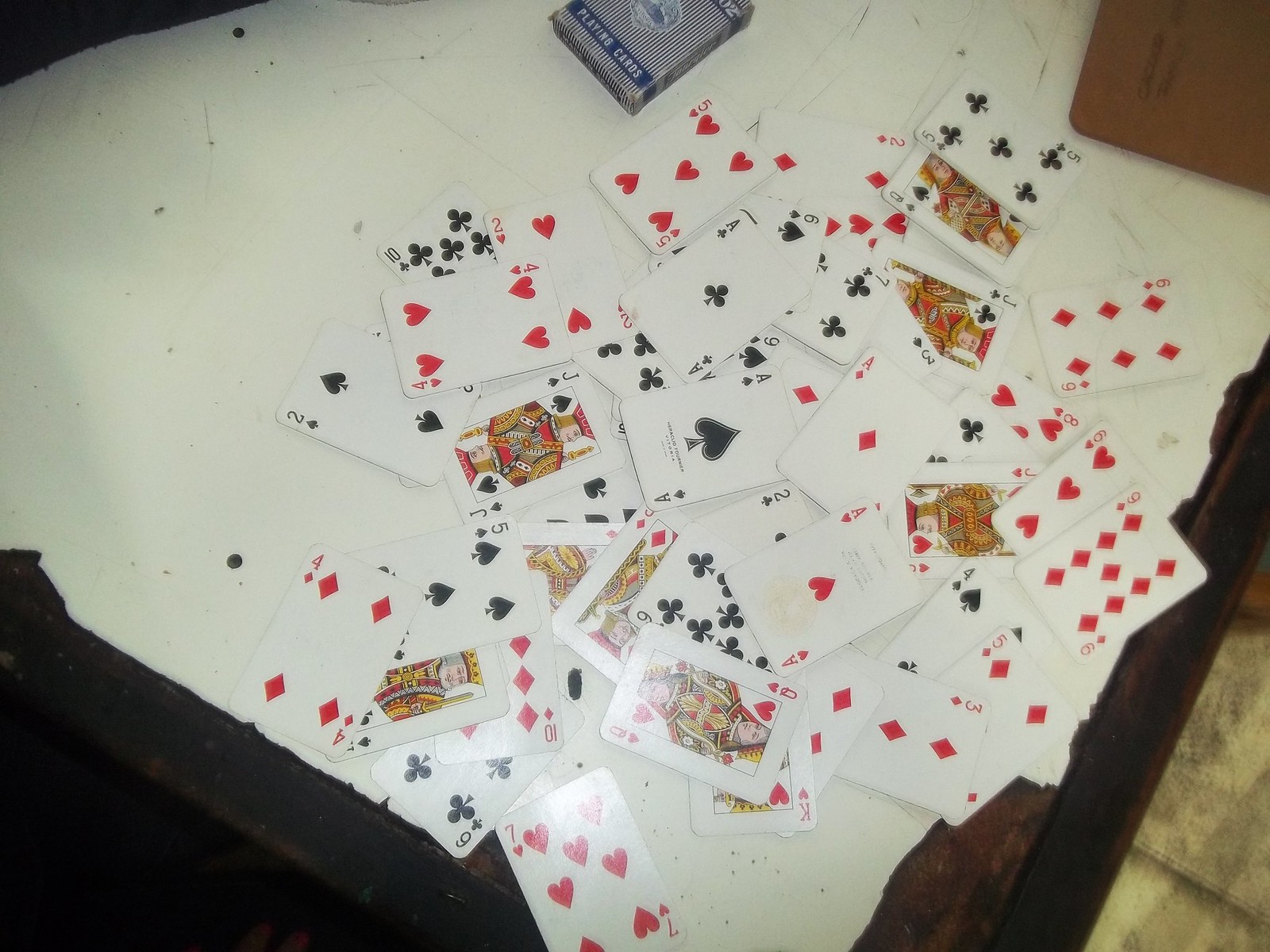A wooden table serves as the base for a visual tableau that captures attention. Atop the table, a large piece of white paper lies haphazardly, its edges jaggedly torn, suggesting a spontaneous or makeshift setup. Spread across this paper in a chaotic yet intriguing manner is an entire deck of playing cards, all face up. Each card displays its number and suit prominently, with enlarged symbols that seem designed for easy readability. 

Near the cards, a box—presumably their container—adds context to the scene. The box is white, alternating with slender blue stripes, and features a blue banner bearing the words "playing cards" in white text. A round logo occupies the center of the banner, but its details remain indistinct. The lower right corner of the image reveals a glimpse of the setting beyond the table, showing a grayish tile floor. This subtle background detail anchors the composition in a casual, everyday environment.